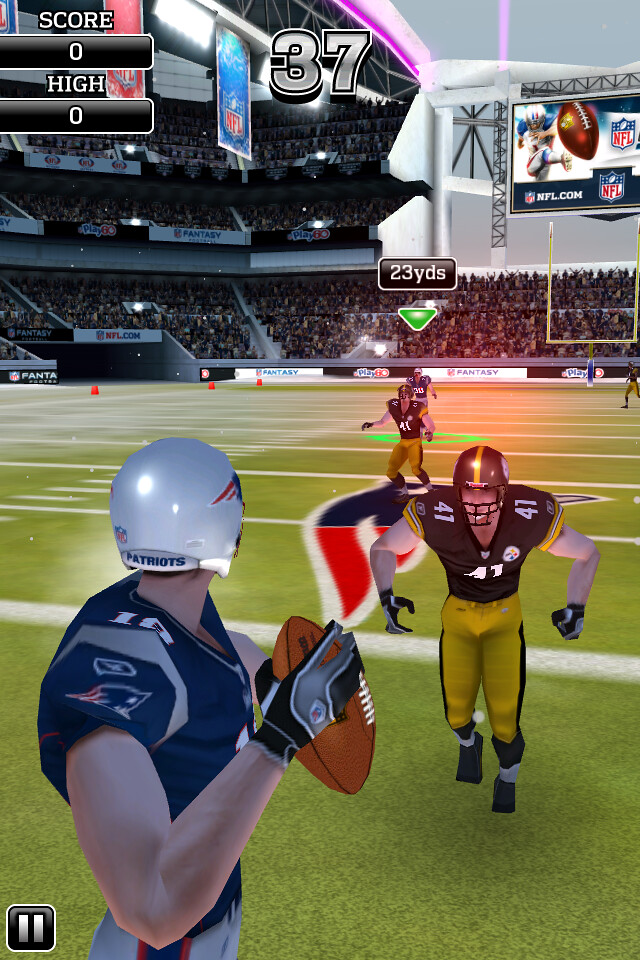In this detailed scene from a football-based video game, the image captures an animated moment on the digital turf. In the top left-hand corner, the screen displays a scoreboard, with the labels "Score" and "High" each followed by black rectangles showing "0". Near the center top, the number "37" is prominently displayed in gray text outlined in black.

Dominating the foreground on the left-hand side, a player donning a white helmet emblazoned with "Patriots" is captured from behind. He stands in a partly sideways stance, clutching the football. To the right, a player in a green jersey with yellow pants faces forward, with an identical teammate positioned directly behind him. The green football field background features clearly marked white yard lines, setting the stage for this intense sports moment.